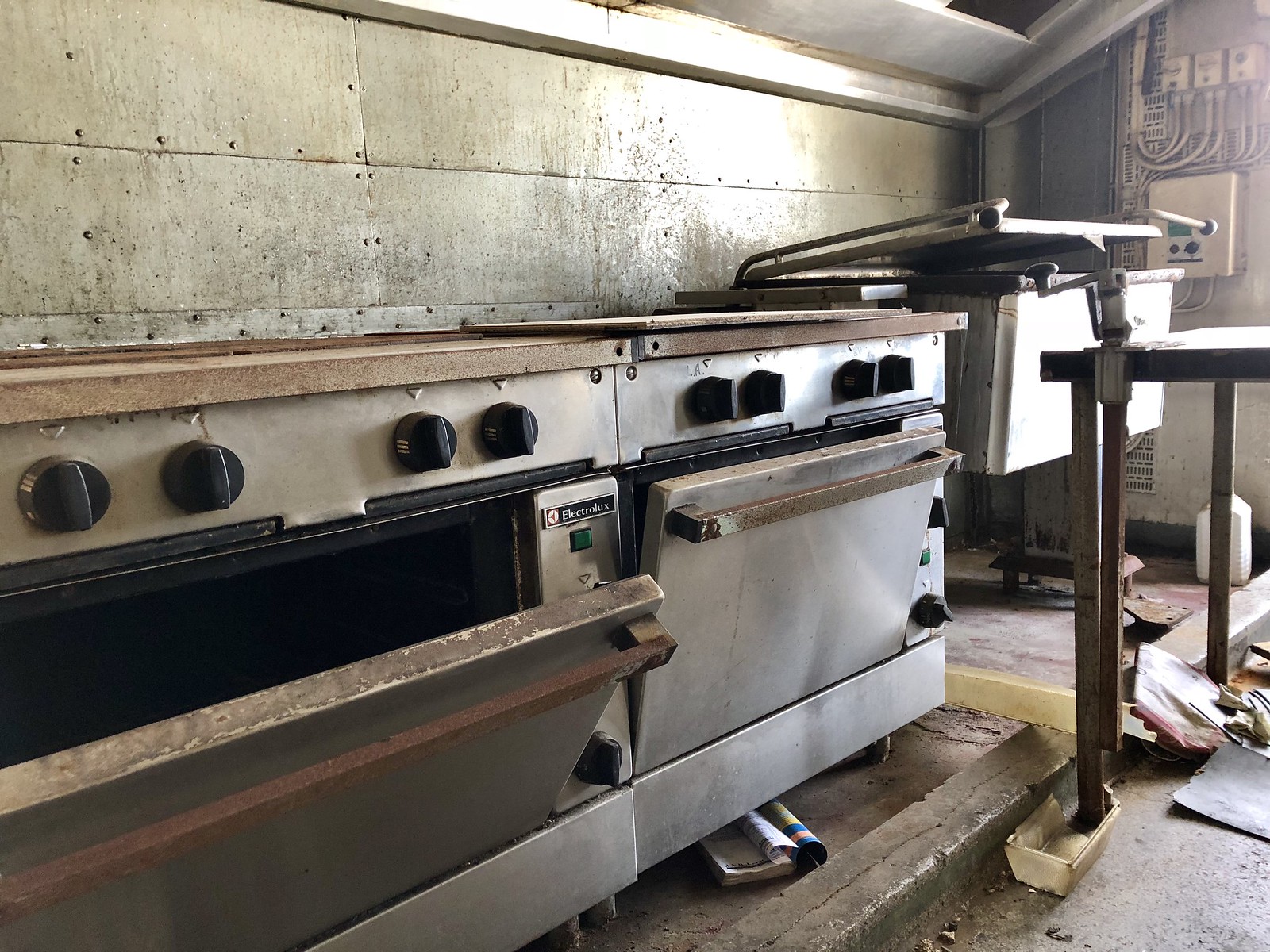This photograph captures an abandoned industrial kitchen likely once used in a restaurant. Dominating the foreground are two large, rusted stainless steel ovens. The oven on the left has its door open at about 30 degrees, while the door on the right is slightly ajar. Each oven features four large black knobs and flat top surfaces, though dirt and rust obscure many details. The concrete floor is littered with debris, including a folded magazine partially tucked under the right oven, plastic containers, and scrap papers. On the far right, a small wooden table, one leg propped on a plastic piece, holds additional miscellaneous items.

The background reveals more about the state of the space: concrete walls with metal panels secured by screws and bolts, and an electrical box connected to smaller electrical components via white wires. Adding to the clutter, there's a plastic jug and what may be a deep fryer or another piece of large metal equipment, its top slightly ajar. The overall impression is of a once-functional kitchen now left to decay, with evidence of heavy use but long-term neglect. Bright light from the left emphasizes the dirtiness and disrepair of the room, highlighting the forlorn ambiance of this abandoned space.